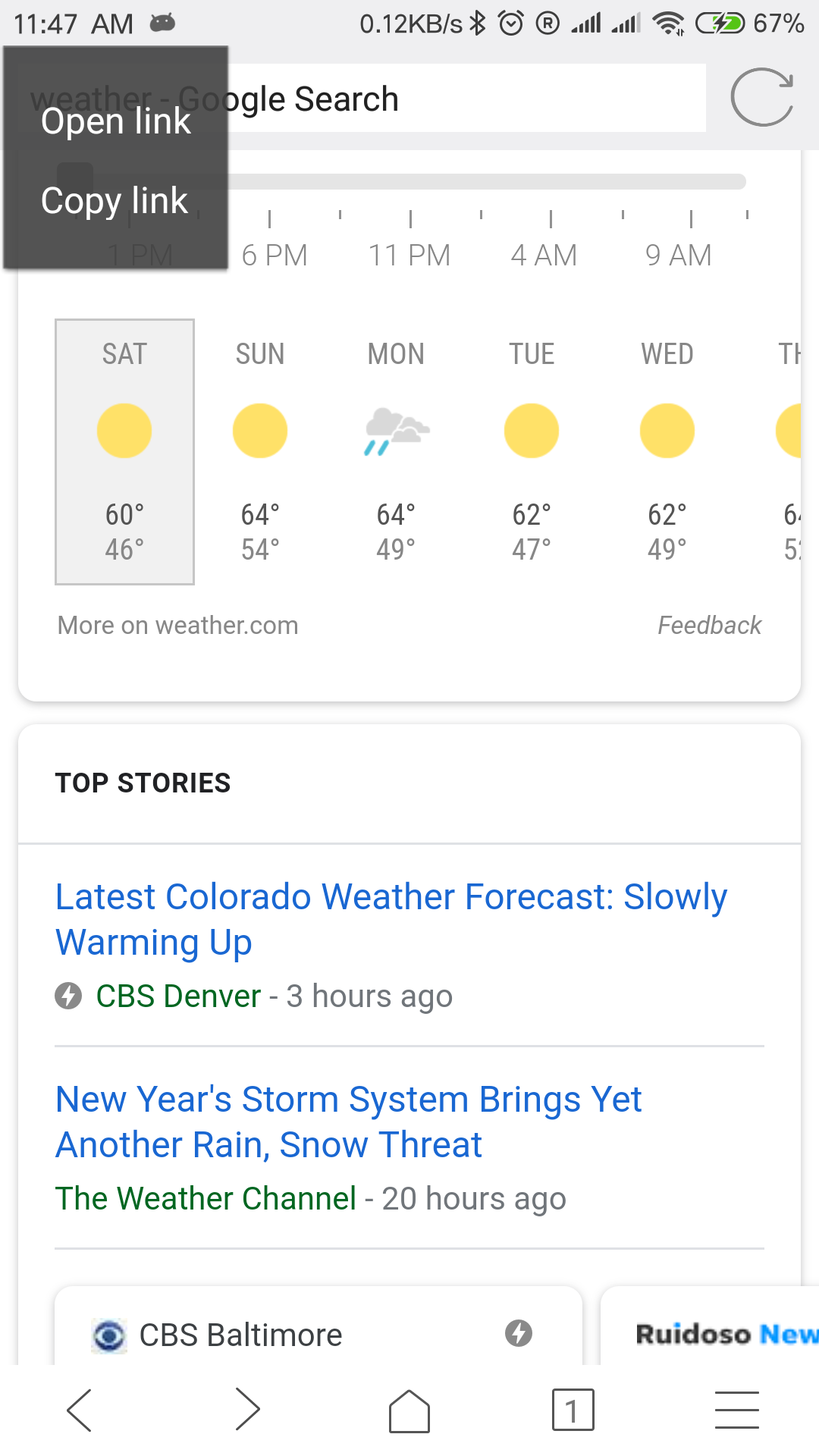A detailed description of the weather information and news page displayed on a cell phone screen:

At the top of the screen, typical cell phone status indicators are visible, including the time "11:47 AM," signal strength bars, an alarm clock icon, Bluetooth and Wi-Fi symbols, and a battery icon showing "67%." Below these icons, a Google search bar contains the text "weather Google search." Overlapping the search bar slightly is a translucent black square with white text options, "Open link" and "Copy link." 

The main content of the page is organized into several sections. The first section displays hourly weather divisions, labeled as "6 PM," "11 PM," "4 AM," and "9 AM." Below these times, the days of the week are listed: "Saturday," "Sunday," "Monday," "Tuesday," "Wednesday," and "TH" (likely an abbreviation for Thursday). Each day has accompanying weather symbols and numbers to indicate the forecast.

Following the weather information, a section titled "Top Stories" appears. The first headline, highlighted in blue, reads, "Latest Colorado weather forecast slowly warming up," with a subtext in black that says "CBS Denver three hours ago." A horizontal line separates this headline from the next. 

The second headline, also in blue, states, "New Year's storm system brings yet another rain snow threat." The subtext, in black, is marked as "The Weather Channel - 20 hours ago." Another horizontal line follows this information.

At the bottom of the page, the CBS Baltimore logo (an eye symbol) is displayed, along with the text "CBS Baltimore," and next to it, a small gray circle featuring a lightning symbol inside. To the right, it says "Roy Dozo, new." 

Finally, navigation icons are shown at the very bottom: a left-pointing arrow, a right-pointing arrow, a house symbol, a square with the number "1" inside, and three horizontal lines stacked on top of each other.